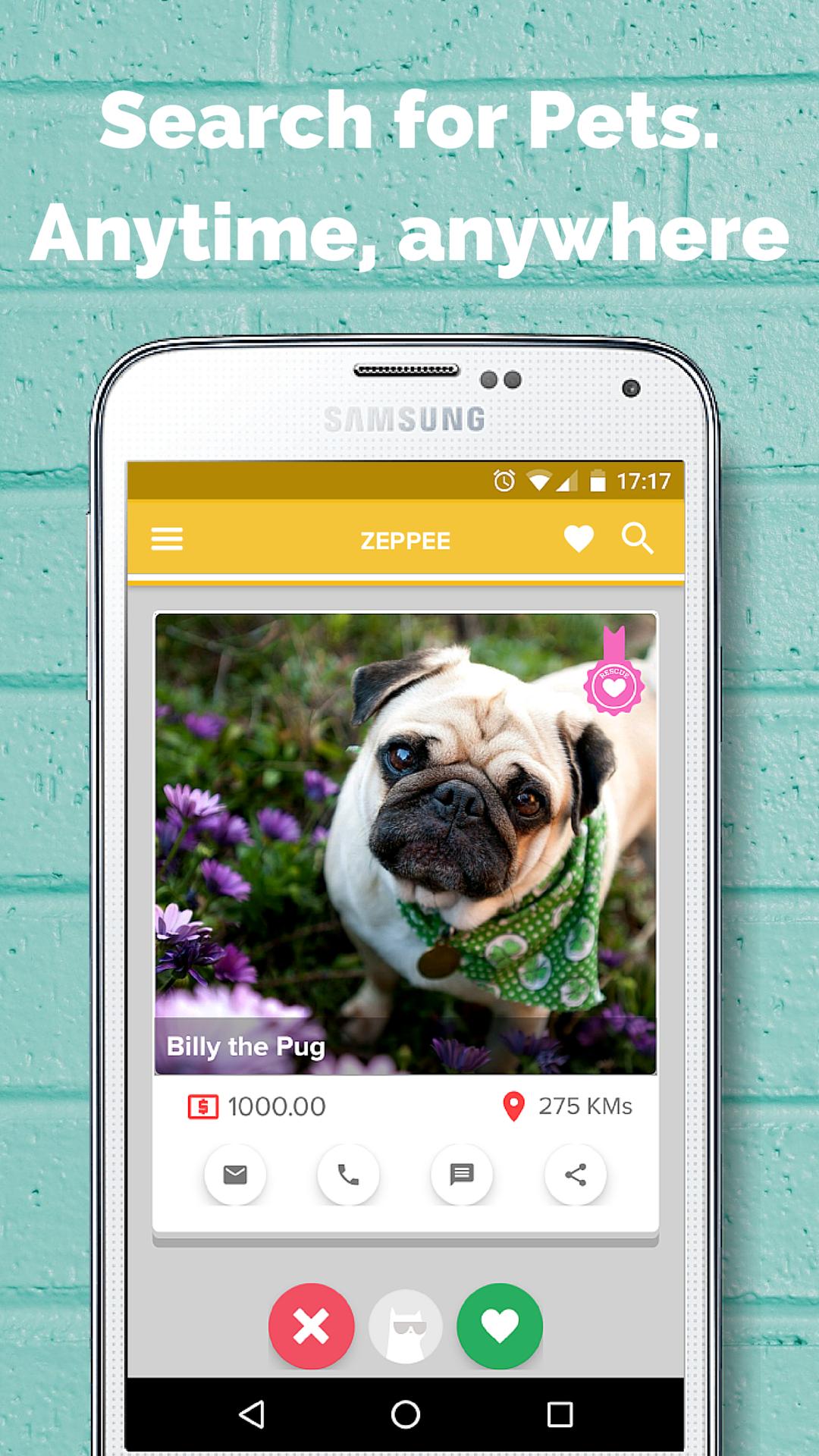The image depicts a vibrant and detailed webpage against a green block wall background with darker green grout. At the top of the page, in prominent white text, it reads: "Search for pets. Anytime. Anywhere." 

Below this banner is an image of a smartphone with a silver outline, showcasing a white background with "Samsung" inscribed at the top. The phone display indicates the time as 17:17, along with a battery icon on an orange line. Directly beneath this, on a dark orange bar, is the text "ZEPPE" in large white letters. To the left of "ZEPPE," there are icons of a heart and a search symbol.

Central to the phone’s display is a photograph of a pug, positioned on the right side of the screen. The pug gazes forward, adorned with a green kerchief around its neck and a round tag on its back. There is also a pink ribbon with a circle bearing a white heart adorning the pug. The dog is predominantly white with contrasting black ears, eyes, nose, and mouth area. Surrounding the pug are purple flowers and green leaves.

To the left of the pug is the text "Billy the Pug," followed by a red dollar sign denoting a price of "1000.00." On the right, it specifies "275 KMS" indicating distance. Below this information are icons for an envelope, a phone, a talk sign, and a share image.

Towards the bottom of the display, there is a red circle with a white "X" and a gray circle featuring a cat wearing sunglasses. Additionally, there is a green circle with a white heart icon.